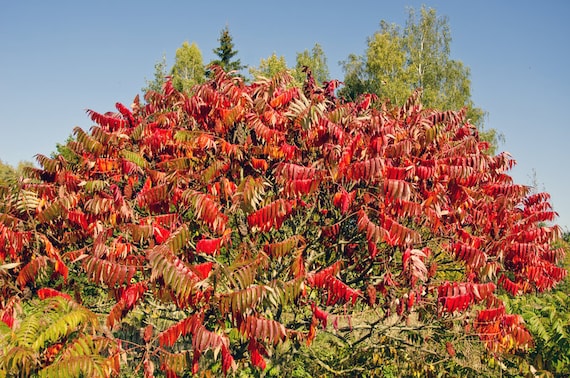The photograph captures a lush, vibrant shrub or small tree adorned with an abundant display of red and orange leaves, suggesting it's either in the midst of autumn or naturally features these colors. Known for its compound leaves where multiple leaflets connect to a single stem, the plant resembles some species of sumac or certain types of ash trees. The shrub, almost mound-like in shape, features a mix of greens and yellows at its base, with green foliage peering through, indicating the presence of other trees or shrubs that haven't turned to fall colors. The background showcases a clear blue sky, enhancing the vivid red, which appears fern-like due to the narrow, side-by-side leaflets or blooms. Contrasting the red leaves is the greenery behind, possibly evergreen trees, creating a striking and colorful natural scene. Additionally, a small-leafed oak tree's tip is visible in the upper right corner, adding to the rich tapestry of foliage captured in the photo.